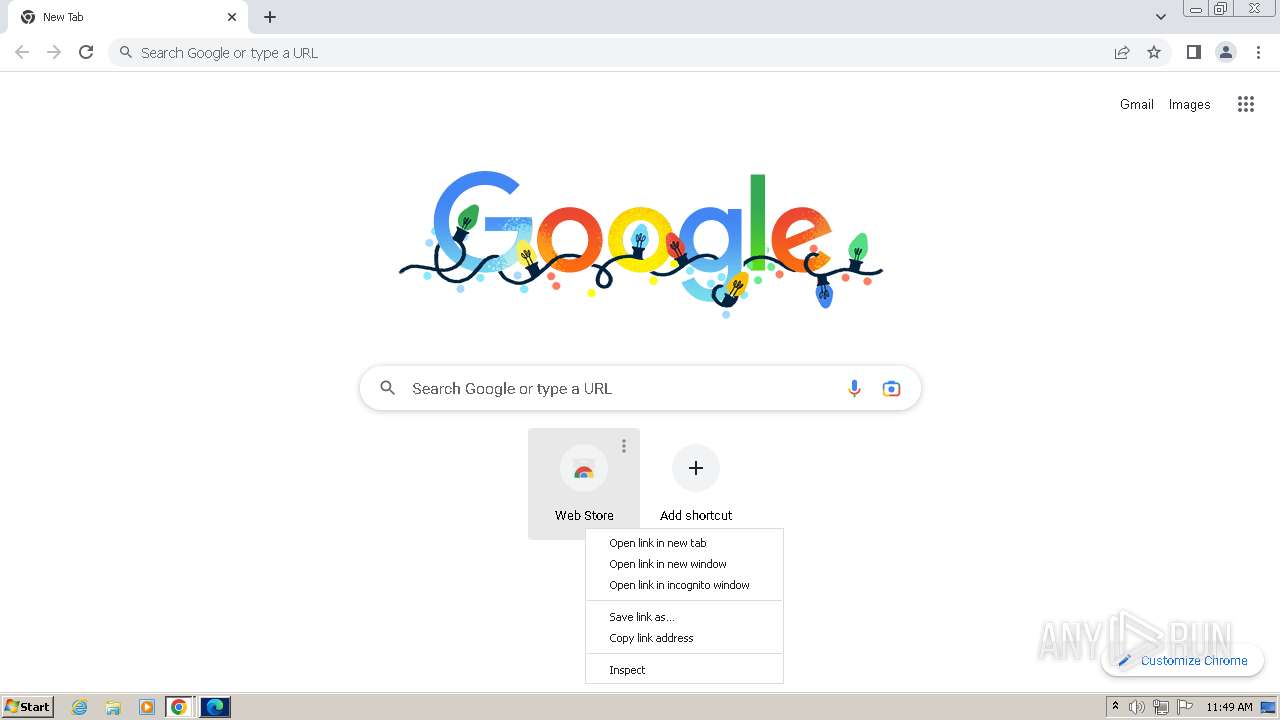The image depicts the homepage of the search engine "Kukli." At the center of the page is the iconic "Kukli" logo, with individual letters styled in vibrant colors: the first 'G' in blue, the first 'O' in red, the second 'O' in yellow, the second 'G' in blue, the 'L' in green, and the 'E' in red. Intertwined with the logo are festive Christmas lights in an array of colors including green, yellow, blue, and red, adding a celebratory touch to the scene.

Beneath the logo, a search bar prompts users with the message "Search Kukli or type the URL." At the bottom of the screen, options titled "Web," "Store," and "Shortcut" are visible for user navigation. Additionally, a context menu has been opened via right-click, displaying commands such as "Open link in new tab," "Open link in new window," "Open link in incognito window," "Save link as," "Copy link address," and "Inspect."

Situated at the top right corner of the page are links labeled "Gmail" and "Images," next to a grid icon signifying the applications menu. On the bottom right, a button marked "Customize Chrome" is present, alongside the current time reading 11:49 AM. The bottom-left corner of the image shows the taskbar of a Windows operating system, with the Microsoft Edge browser icon, Chrome, Windows Media Player, File Manager, and Explorer visible, as well as the Start menu button.

In the lower section of the image, a subtle watermark reads "Any Run" in grey text, indicating the context or tool used for capturing or analyzing the image.